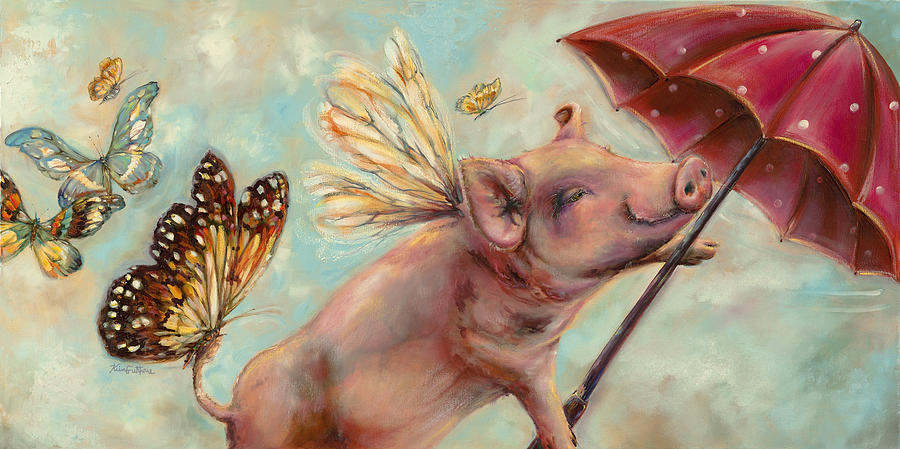This captivating painting, set against a soft blue sky with hints of peach-colored clouds, features a charming piglet at its heart. The piglet, depicted with closed eyes and a joyful smile, seems to hover in mid-air thanks to its delicate fairy-like wings and a whimsical addition of a bright red umbrella with white polka dots clasped between its front hooves. Surrounding this fantastical scene are a series of beautifully vibrant butterflies in hues of blue, orange, green, yellow, and more. Most strikingly, one large butterfly with orange-tipped wings and white polka dots appears to be aiding the piglet’s flight by gently holding its tail. Additional butterflies, including a tiny light green one above the piglet and others with varied colorful patterns, flutter gracefully in the backdrop, enhancing the enchanting atmosphere of the painting. The artwork is completed with a barely discernible signature below the butterfly holding the piglet's tail, underscoring the professional quality of this delightful and imaginative piece.